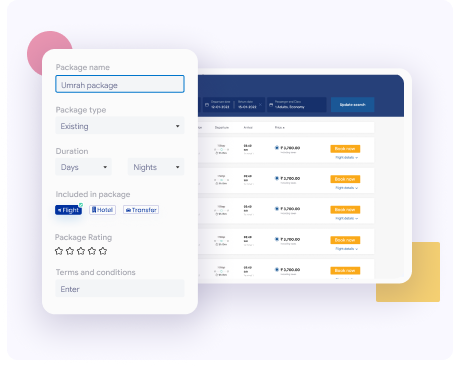The image features a light gray background with a purple circle located in the top-left corner. A rectangular shaped pop-up dominates the center of the image, oriented vertically.

At the top of the pop-up, in gray text, "Package Name" is written. Directly below it is a text box bordered in light blue, containing the words "Oomera Package." Beneath this text box, the label "Package Type" is displayed, followed by a drop-down box labeled "Existing."

Continuing downward, the next section is labeled "Duration." Here, there are two drop-down boxes side-by-side: the left one is labeled "Days" and the right one is labeled "Nights."

Following the duration section, the text "Included in Package" is presented. Under this, there are three buttons labeled "Flights," "Motel/Hotel," and "Transfer," respectively.

Further down, the text "Package Rating" appears, along with a section featuring five stars for rating purposes. However, none of the stars are highlighted or lit up.

At the bottom of the pop-up, the words "Terms and Conditions" are displayed, accompanied by an "Enter" button.

In the background, which is somewhat blurred and small, there are various pieces of flight information, including prices and other travel-related data.